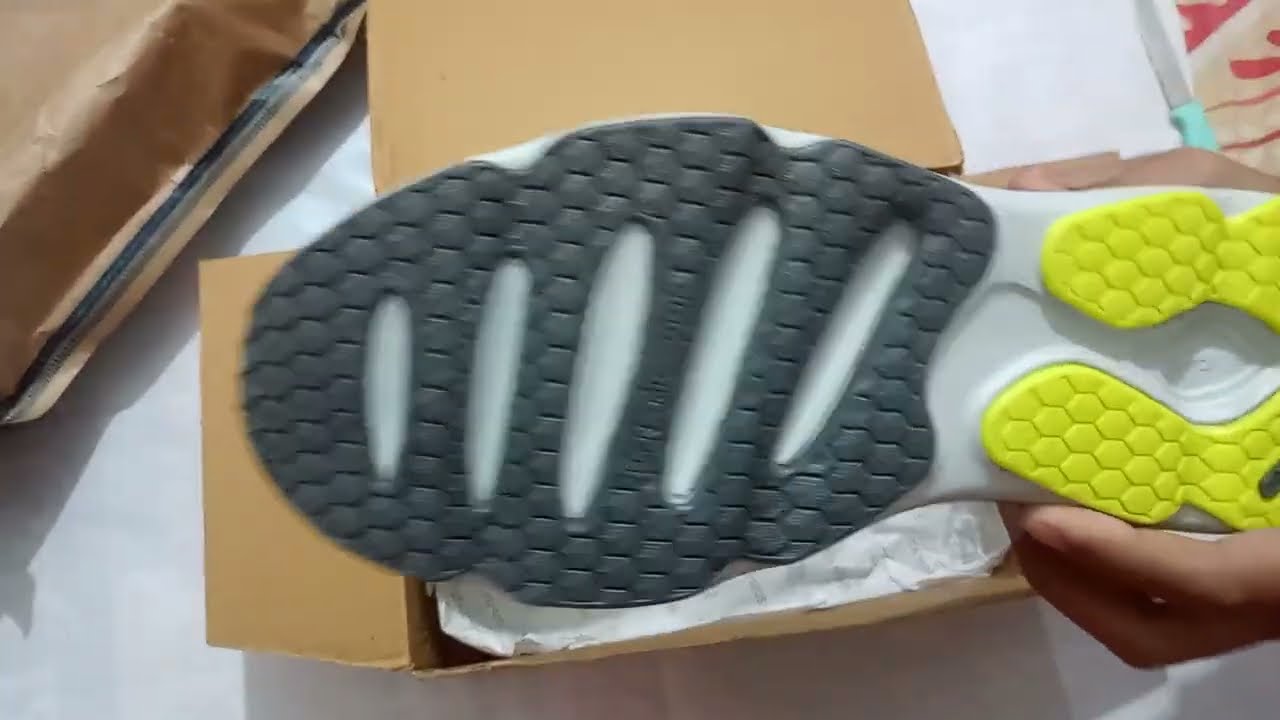The image depicts an unboxing scene where a person with darker skin is holding up the left shoe, displaying its sole prominently. The shoe is oriented sole side up, with its toe pointing towards the left and the heel, partly out of the frame, towards the right. The image is a bit blurry, possibly due to the person's excitement while unboxing. The sole of the shoe is primarily white with distinct black grips at the front and yellow grips near the ankle area. The shoe also features a fluorescent greenish-yellow wavy pattern along the bottom, resembling a horseshoe at the heel. In the background, an open shoe box with white tissue paper is visible, alongside some packaging remnants on the upper left.